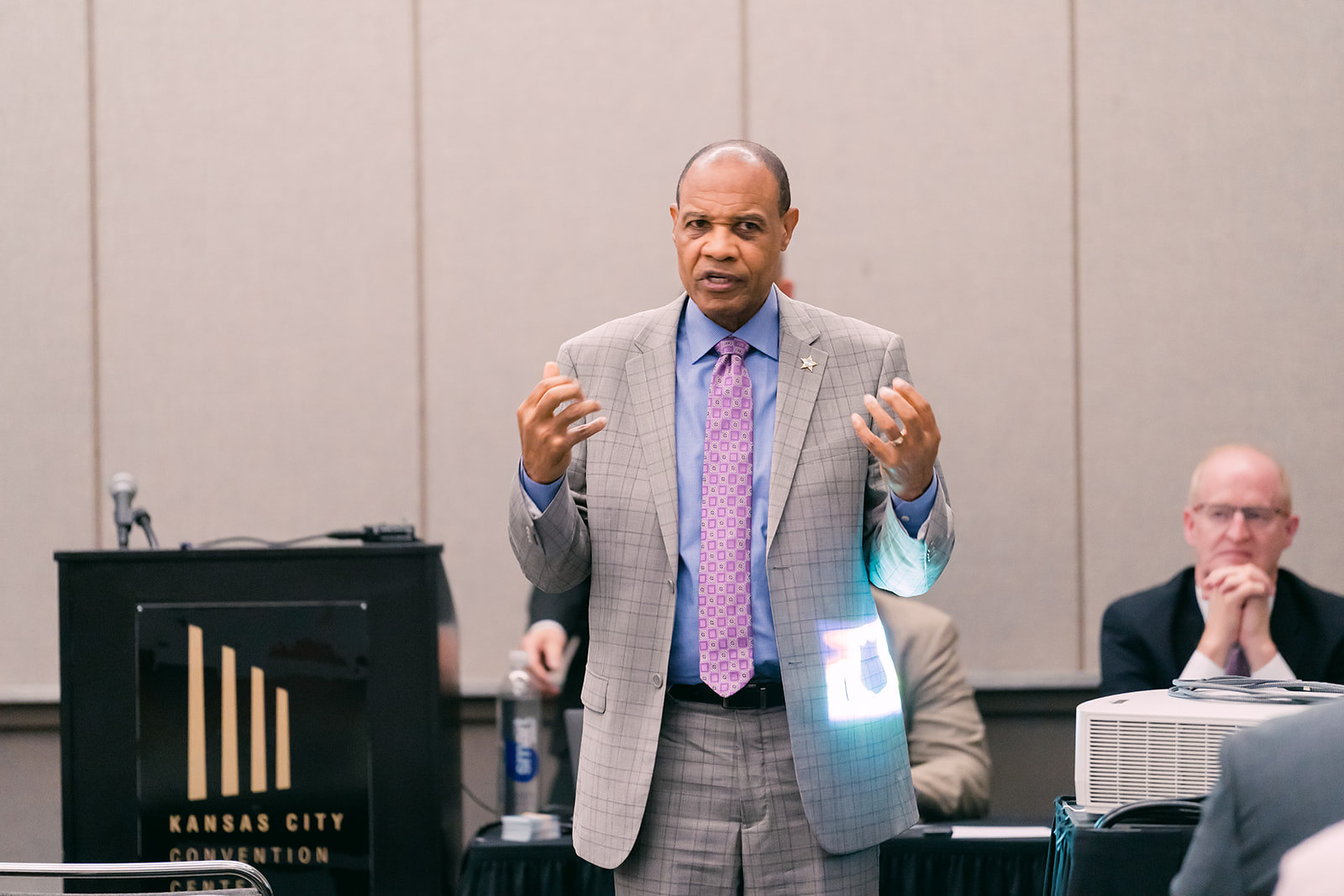In this horizontally aligned rectangular photograph, a man stands at the center, evidently delivering a speech at a formal event. He is predominantly bald with very short black hair and is clad in a striking gray plaid suit paired with matching pants. His outfit includes a light blue button-down shirt and a light purple-patterned tie, which complements his attire. The man's left pocket on his suit jacket appears to be illuminated, and he is positioned with his hands raised in front of him, fingers slightly curled, seemingly gesturing as he speaks with his mouth open.

To his left, a black podium adorned with vertical gold bars stands prominently. It bears the inscription "Kansas City Convention Center" in gold text and is equipped with a silver microphone. Behind the speaker, on his right, another older man with very short white hair and glasses watches intently. He appears partly bald, wearing a black suit and white shirt, and has his hands clasped under his chin. Only the side of a third man's suit jacket is visible directly behind the speaker.

The background consists of large vertical beige-colored slats, suggesting the setting is within a conference room or similar formal venue. The photograph captures the essence of the event, highlighting the primary speaker in his detailed, formal attire against the structured, professional backdrop.